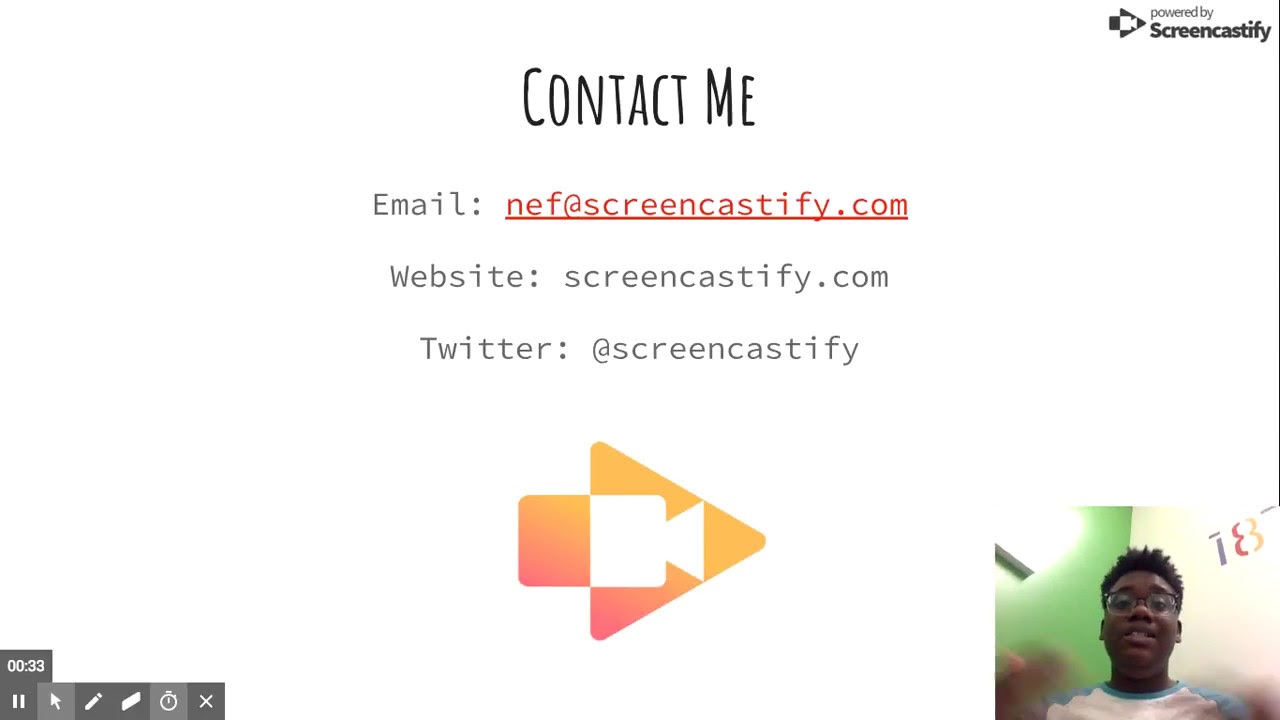The image features a "Contact Me" page, prominently displayed in the center, displaying the following details: 

- "Contact me" at the top.
- Below it, the email: "nef@screencastify.com" in red text.
- The website: "screencastify.com"
- Twitter handle: "@screencastify."

In the lower portion of the image, an arrow icon with an orange-red gradient background and a white camera logo is visible. The top right corner of the image is branded with "Powered by Screencastify." 

The bottom right corner showcases a young black male, viewed from what appears to be a webcam screenshot. He wears glasses and a white t-shirt with blue accents. His hair is short, and the wall behind him is a combination of green and white, bearing the number 18. 

There are also slideshow controls visible in the bottom left, including buttons for pause, arrow, right, erase, timer, and exit, labeled "0033."